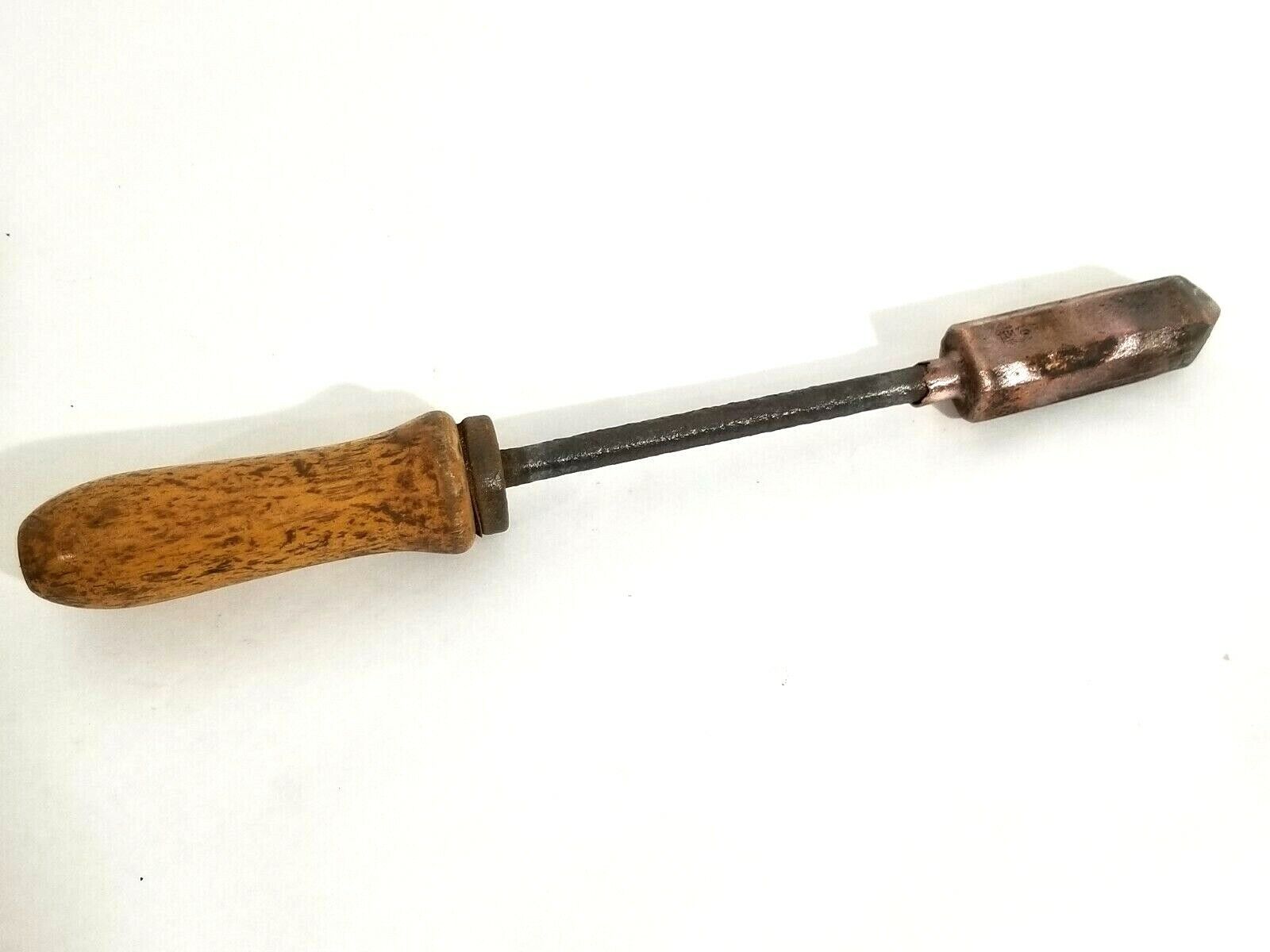The image depicts an old, well-worn tool, likely an ice pick or hole punch, lying horizontally on a white, blank surface. The tool features a rounded, brownish-yellow wooden handle that appears very aged and used, reminiscent of a rolling pin handle. Connected to the handle is a cylindrical flat metal piece, resembling a washer or nut, which is slightly rusted. Extending from this metal piece is a long, thin cylindrical rod that appears to be blackened with dirt or grease but not rusty. At the far end of the rod, there is a robust club-like metal appendage featuring a cylindrical section leading to a long, rectangular part that tapers into a fine point. The background is stark white, accentuating the tool's shadow, and there is nothing else in the photograph to distract from the image of the tool.